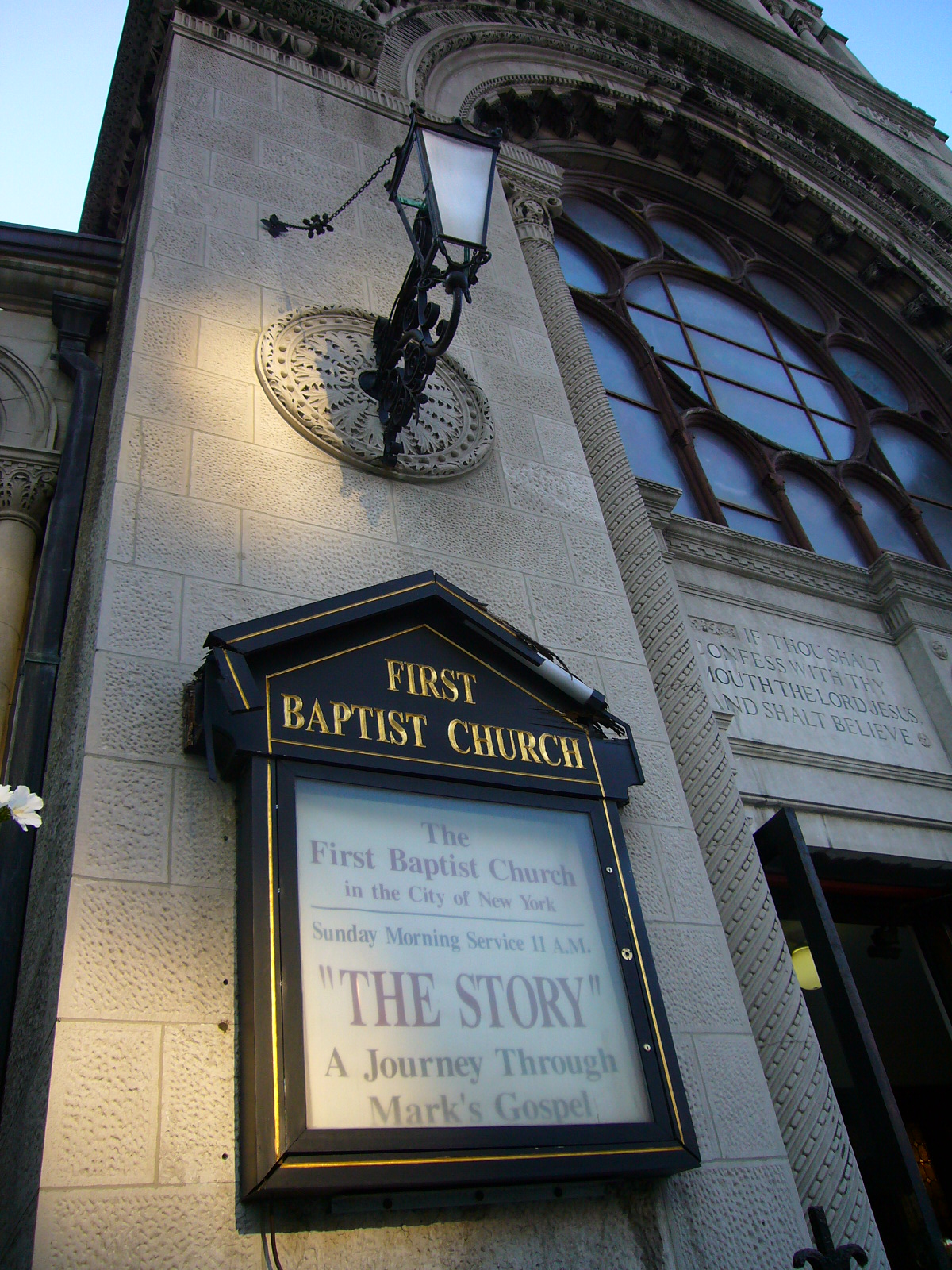The image depicts the facade of the historic First Baptist Church in New York City, captured from an upward angle. The building is constructed from tan stone, giving it an old and ornate appearance. A portion of the sky is visible at the top edges of the photo, adding a touch of blue to the scene. 

At the top of the image, a black sconce with white coverings is mounted on the wall, showing signs of wear with splintering wood. Directly beneath the sconce is a house-shaped sign marked with gold detailing and the text "First Baptist Church" at the top. Beneath this, another section of the sign announces in alternating red and black fonts: "The First Baptist Church in the City of New York. Sunday morning service 11 a.m. 'The Story,' A Journey Through Mark's Gospel."

To the left, a spoke-shaped brownish window with multiple circular modules is a highlight of the architectural design. Additionally, partially visible at the bottom left of the image are the dark-colored main doors of the church, which are slightly ajar. Above these doors, there is an engraving that reads, "If thou shalt confess with thy mouth the Lord Jesus, and shalt believe." The overall composition of the photograph effectively showcases the church's intricate and historical architecture, albeit no people are present in the scene.